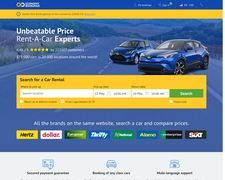The image depicts a website interface dedicated to car rentals. At the top, there is a chain icon and a blue bar with text that reads "Unbeatable Prices" and "Rent-A-Car Experts." The centerpiece of the image features two blue cars on an asphalt road, flanked by grass on either side. Road lines are visible, adding to the authentic roadway appearance.

Below this scene, the website offers a search bar for users to enter information to find car rentals. There are sections for selecting car brands, with logos of notable companies such as Hertz, Dollar, and Thrifty displayed, although they appear quite pixelated. Additionally, there is a green square highlighting the message "All the brands on the same website," emphasizing the site's comprehensive rental search capability.